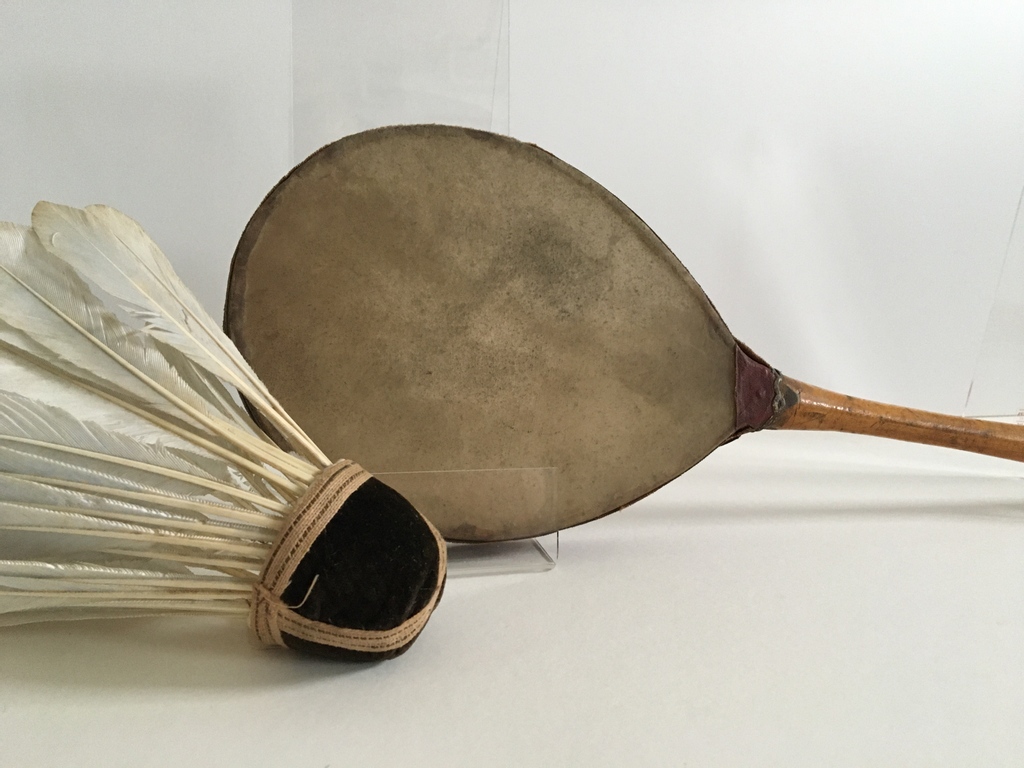This close-up photograph captures a set of very vintage badminton equipment displayed against a stark white background. The centerpiece is an aged badminton racket with a light-colored wooden handle, positioned vertically with its handle angled slightly to the right. The head of the racket is encased in a mottled, dark brown, and very worn leather cover. To the left lies a genuine feathered shuttlecock, its leather-trimmed end point facing left and showcasing tan rawhide strips wound around a black head. Both items cast soft shadows on the white table, highlighting their aged textures and historical significance.